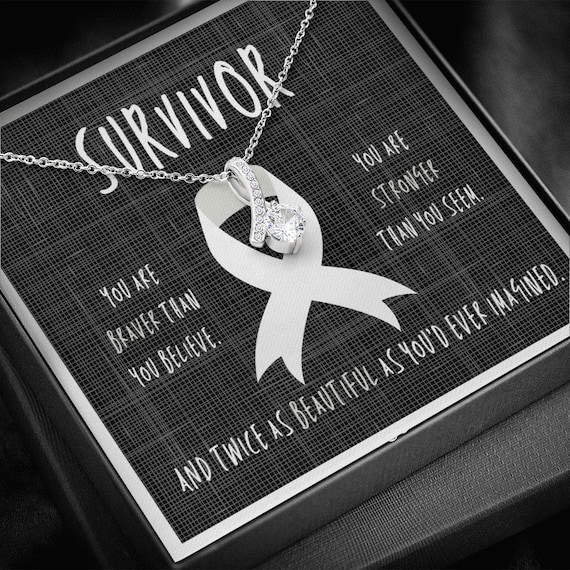This black-and-white photograph captures an elegant necklace displayed in an open jewelry case. The necklace features a silver chain adorned with a large central diamond that swirls into a ribbon shape studded with smaller diamonds. The design prominently includes the breast cancer awareness ribbon motif. The necklace is laid out on a fabric platform inside a textured, black box, which is outlined in white and crisscrossed with thin white lines. The box includes an inspirational inscription that reads: "Survivor. You are braver than you believe, you are stronger than you seem, and twice as beautiful as you'd ever imagined." The ends of the chain extend towards the top corners of the box, suggesting their continuation behind the platform. The entire scene is set against a black background, emphasizing the elegance and emotional message of the jewelry.